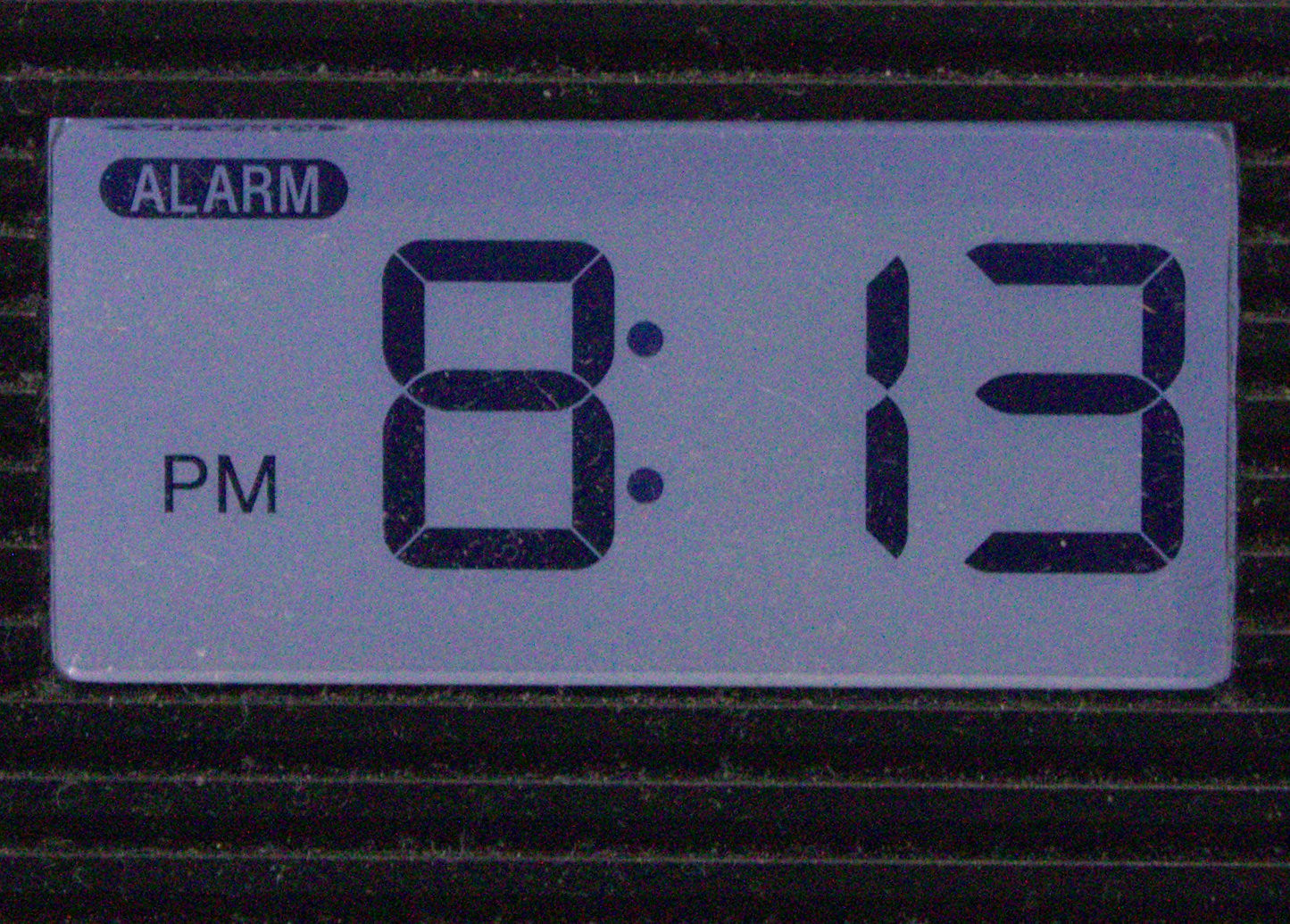A detailed close-up photograph of a digital alarm clock face. The screen, tinted in a blue-grayish hue, prominently displays the time as 8:13 PM in standard black digital font. In the upper left corner, an alarm icon, enclosed in a black oval, signifies that the alarm is set. Surrounding the screen is a black plastic casing, featuring several horizontal lines with indentations, giving it a textured appearance. Dust has collected within these indentations, highlighting the clock's worn, slightly neglected state.